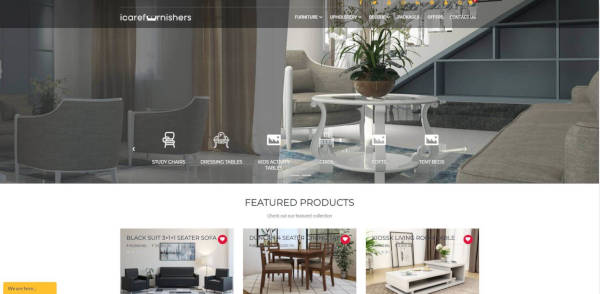This appears to be a screenshot of a furniture company's website. The header prominently features the company name "I Care Furniture," creatively designed with the silhouette of a tiny couch replacing the letter 'U' in "Care." The navigation bar has several tabs, though only the 'Furniture' tab is discernible due to its clarity; the other tabs are blurry and hard to read.

Below the header, there's a serene image of a home interior showcasing a gray and white color scheme. The space features a white side table, sandy-colored chairs, and a matching sandy-colored couch, presenting a cohesive and inviting atmosphere.

Scroll down to the "Featured Products" section, where three images are displayed:

1. **Black Suede Three-Seater Sofa**: This deep charcoal, almost black, sofa is a striking centerpiece. The sofa is flanked by two single chairs, creating a cozy, stylish arrangement.
   
2. **Dining Table with Four Chairs**: A robust, rectangular table with a rich, dark red-brown wood finish is accompanied by four chairs. The chairs feature deep sandy-colored seat cushions, adding both comfort and a hint of contrast to the dark wood.

3. **Modern, Multifunctional Coffee Table/Display Unit**: This unique piece could serve as either a coffee table or a TV display unit. It has a rectangular surface that extends over a more square one, both featuring built-in storage holes for added functionality and a contemporary aesthetic.